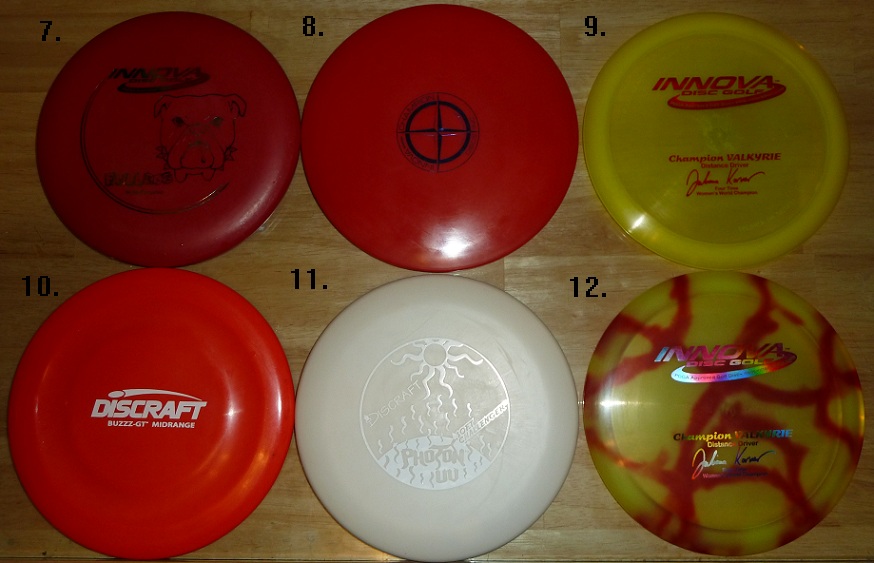The image displays six frisbees arranged in two rows of three on what appears to be a wooden or laminate surface. Each frisbee is accompanied by a black number, ranging from 7 to 12, positioned just above the top-left side of each. In the top row, the first frisbee on the left is red and features an image of a bulldog with the number 7 above it. The second frisbee is also red and displays a compass emblem in black, indicating directions with the number 8 above it. The third frisbee is yellow with the word "Innova" written in red, marked by the number 9. In the bottom row, the first frisbee is bright red with the word "Discraft" printed on it in white, accompanied by the number 10. The middle frisbee in this row is white, showcasing an engraving of a sun, and is numbered 11. The final frisbee on the right is yellow with abstract red streaks, also bearing the word "Innova" in iridescent writing, numbered 12.